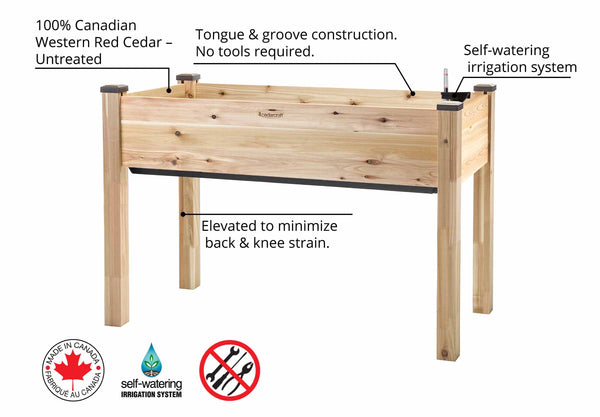The image depicts an elevated wooden planter that resembles a table, constructed from 100% Canadian Western Red Cedar, untreated. The planter features four long legs and an open top resembling a box that is about five inches deep, with dimensions approximately a couple of feet long and a foot or so wide. The wood is described as having a light oak appearance and utilizes a tongue and groove construction, which means it can be assembled without tools. The planter is designed to minimize back and knee strain by elevating the planting surface. It is equipped with a self-watering irrigation system, indicated by a label featuring a water droplet. Additional labels highlight its Canadian origin, with a circle containing a red maple leaf and the text "Made in Canada." The image background is white, providing a clear view of the product and its descriptive text.